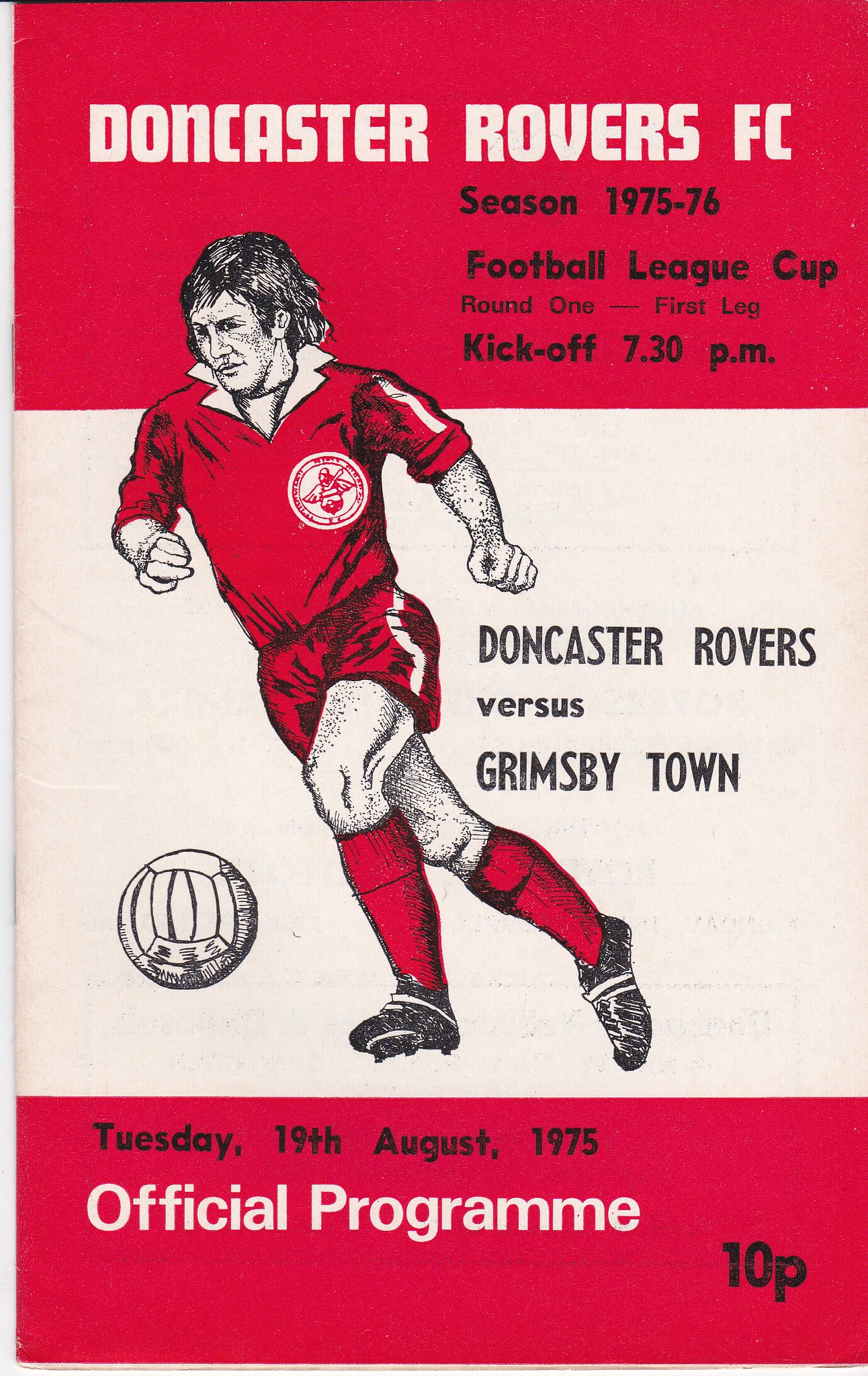The image is the front cover of an official soccer program for a sporting event. At the top, in white letters against a red background, it reads, "Doncaster Rovers FC season 1975-76 Football League Cup Round One First Leg Kickoff 7:30 p.m." Below this, the text continues, "Doncaster Rovers versus Grimsby Town, Tuesday 19th August 1975, official program 10p." The center of the image features a cartoon drawing of a soccer player, dressed in a red uniform with a white collar and white stripe down the sleeves. The player is kicking a soccer ball, and the entire illustration is rendered in shades of white, black, red, and gray. The player wears red shorts with a white stripe on the side, red socks, and black shoes.